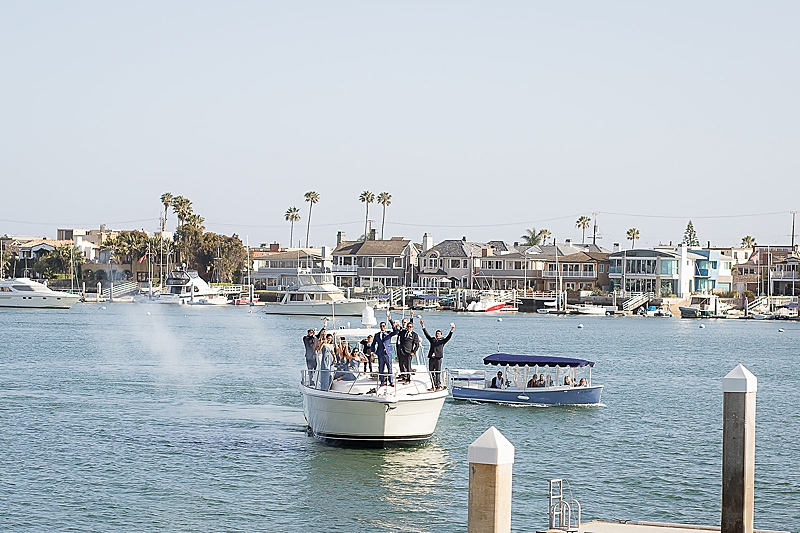Set against a hazy gray sky in what appears to be a tropical harbor, this detailed scene captures a bustling marina with numerous boats and a backdrop of elegant two- and three-story houses. Central to the image is a white cabin cruiser on the left, marked by a black trim at the bottom and a silver-colored barrier around its edge. The boat is teeming with people, featuring a mix of men in suits and women in long gowns, some raising their glasses as if toasting—a lively scene that might suggest a celebration or wedding party. Prominently, one individual in a black shirt and another in a blue suit stand out, while a young lady in a light blue dress is seen reclining. To the right of this main boat is a smaller vessel adorned with a dark purple canopy supported by white bars; this ferry-like boat with several seated individuals seems poised to dock. Further to the left on the water, a sleek yacht with a slanted back windshield makes its appearance, emitting light smoke. The water, rippling gently in a light gray hue, is dotted with reflections of the surrounding activity, while palm trees in the distance hint at a coastal, possibly West Coast or tropical, locale. The foreground features a dock equipped with posts and a ladder descending into the water, anchoring this vivid maritime tableau.